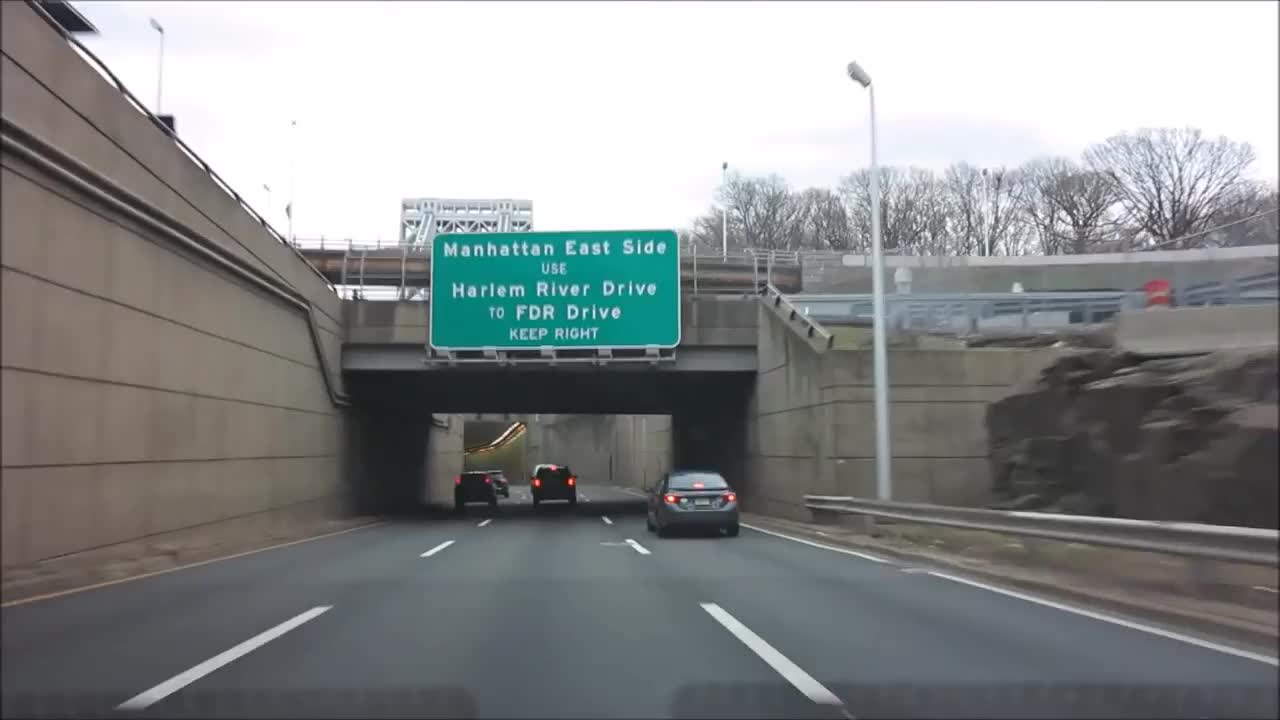The photograph, taken from inside a moving car, captures the view through the front windshield with a slight glare and part of the dashboard visible. The car is traveling down a three-lane road with white dashed lines marking the lanes. Ahead, multiple cars with their red brake lights or taillights lit up are seen, spaced out by a few car lengths. The road is leading into a tunnel or a bridge area that is covered. On either side of the road, there are several stories high concrete walls. Above the overpass, an illuminated green directional road sign reads "Manhattan Eastside. Use Harlem River Drive to FDR Drive. Keep right" in white reflective text. Street lights dot the path, and inside the tunnel ahead, additional overhead lights are visible, guiding vehicles through the covered structure.